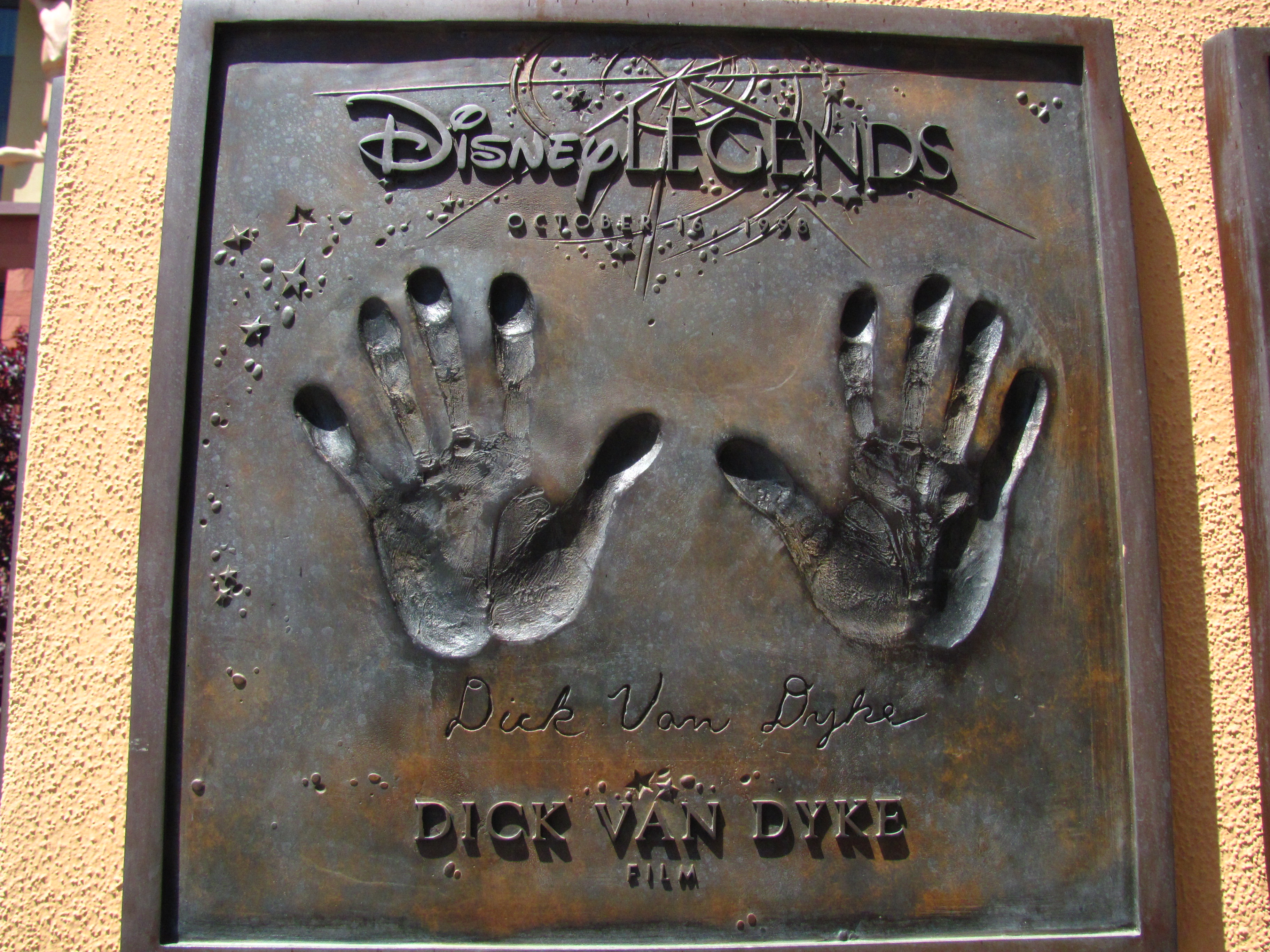The image depicts a bronze-colored metal plaque with two hand imprints, one of a left hand and one of a right hand. This plaque is mounted on a yellow, bumpy-textured wall. The plaque features a raised edge that frames the entire piece, which is detailed with multiple lines of raised text. At the very top of the plaque, it reads "Disney Legends," with a design of multiple stars swirling above this text. Centrally positioned on the plaque are the aforementioned handprints. Directly below the hand imprints is a cursive autograph that reads "Dick Van Dyke." Beneath the signature, the name "Dick Van Dyke" is also printed in standard font, followed by the word "Film" in smaller font at the very bottom. The colors in the image vary, showcasing shades of bronze, rust brown, and hints of tan and black, with a splash of light-colored pink visible on the left side. The photograph appears to have been taken at an angle, focusing downwards onto the plaque, capturing the details and textures vividly.